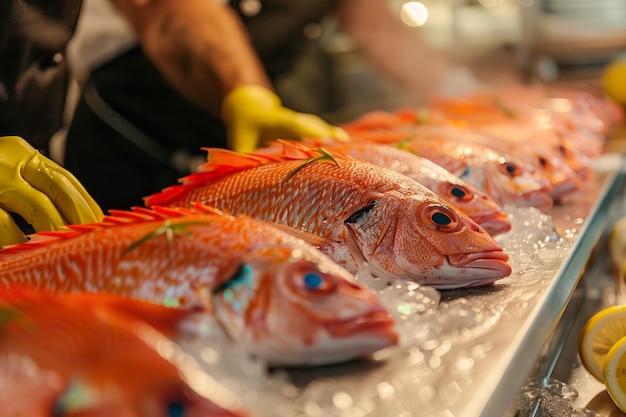In this color photograph of a fish market, a long, silver tray filled with ice features prominently, extending from the bottom left to the top right of the image. Resting on this tray are several dead fish, possibly salmon, with scales that are bright orange and bodies that are light orange with pinkish speckling. The fish in the middle are the clearest, while those closest and furthest are slightly blurred. To the left side, a pair of tattooed hands wearing yellow latex gloves are seen handling two of the fish, suggesting they are preparing or arranging them. The person appears to be wearing a black apron over a white shirt. In the background, another person can be seen, although more blurred, also wearing yellow gloves. On the right side of the counter, two sliced lemon wedges are visible. The overall setting suggests an outdoor or street fish market, with the focus on the fresh display of fish ready for sale.